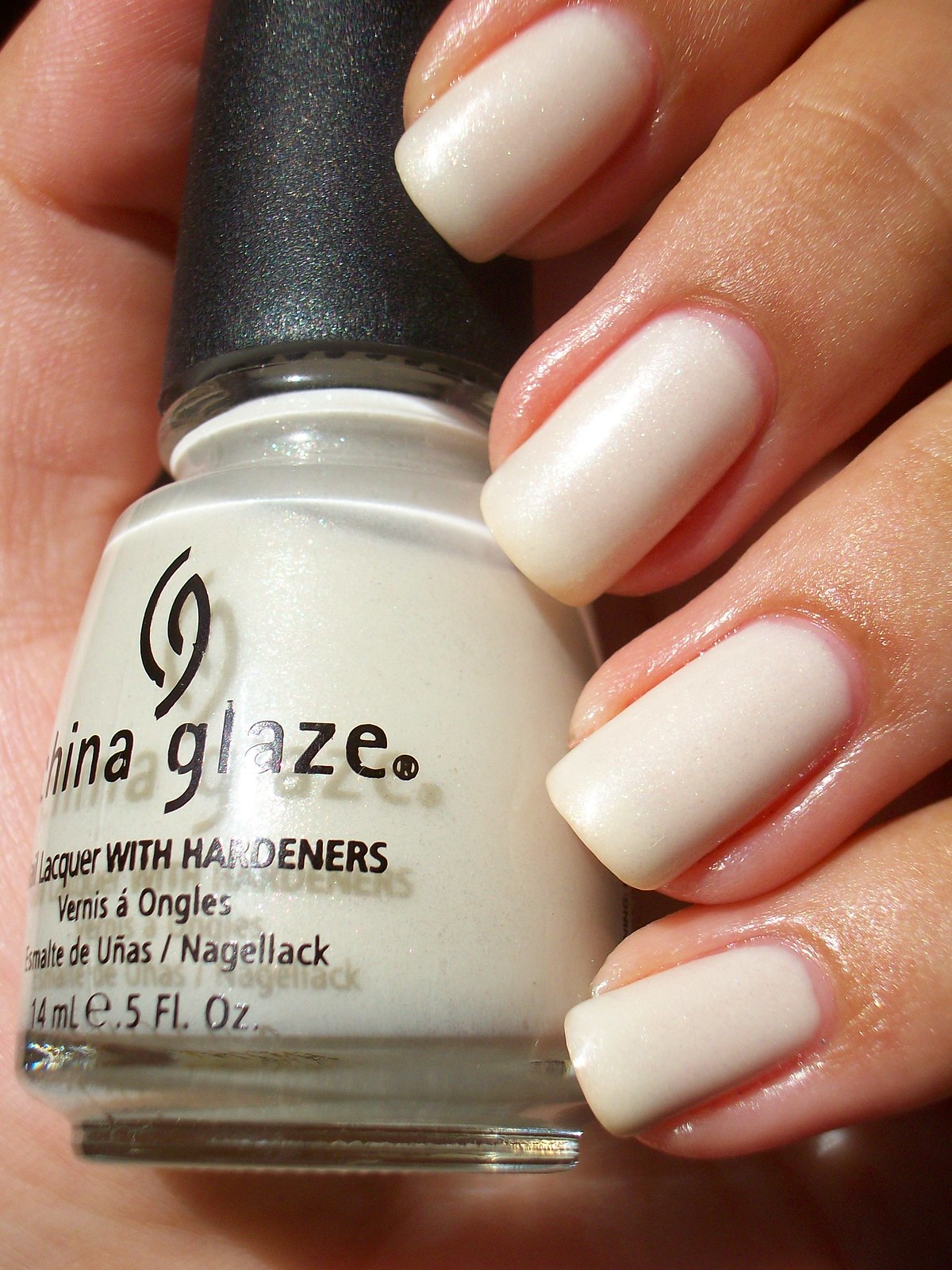The image features a frosty white bottle of nail polish with black text branding that reads "China Glaze Lacquer with Hardeners." The bottle sports a sparkly black lid and contains five fluid ounces of polish. The intricate logo resembles a vertical eye or flame. Positioned centrally in the frame, the bottle is held in the palm of a hand, with only the fingers and freshly painted nails visible. The background consists mainly of the person's hand, creating a close-up and intimate setting. The polished nails match the color of the nail polish in the bottle, suggesting a recent application. The scene appears to be a review or promotional photograph of the nail polish, with a color palette including black, tan, white, pink, and gray tones.